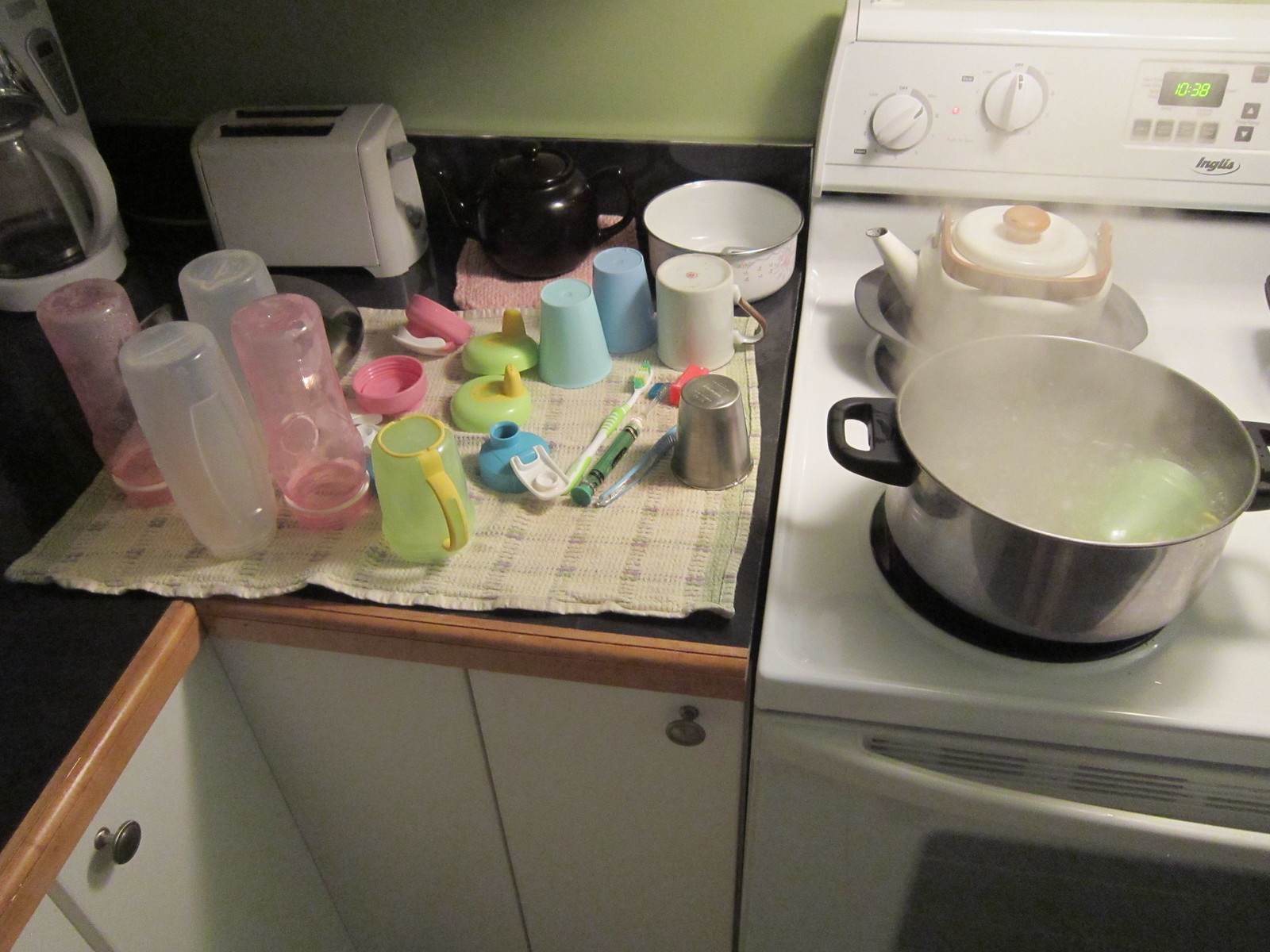A detailed view of a kitchen stove reveals a bustling scene of sterilization. The white stove, featuring a dial with green digits reading "1038," displays the INGLIA logo in gray at the base. A large silver pot with black handles is perched on a burner, its contents boiling vigorously. Curiously, a plastic cup bobs in the boiling water. Beside it, a tea kettle with a white body and brown handle occupies a second burner, with a metal pan underneath.

To the left, a black kitchen surface with wood accents is visible, adorned with a neatly laid checkered towel in white and light purple. Various items suggest the process of sterilizing baby equipment: baby bottles, sippy cups, toothbrushes, a medication syringe, and a coffee cup are all present. The colorful assortment of baby cups in greens, blues, and pinks adds a vibrant touch to the scene, indicating a practical yet chaotic moment of thorough cleaning and sterilization.